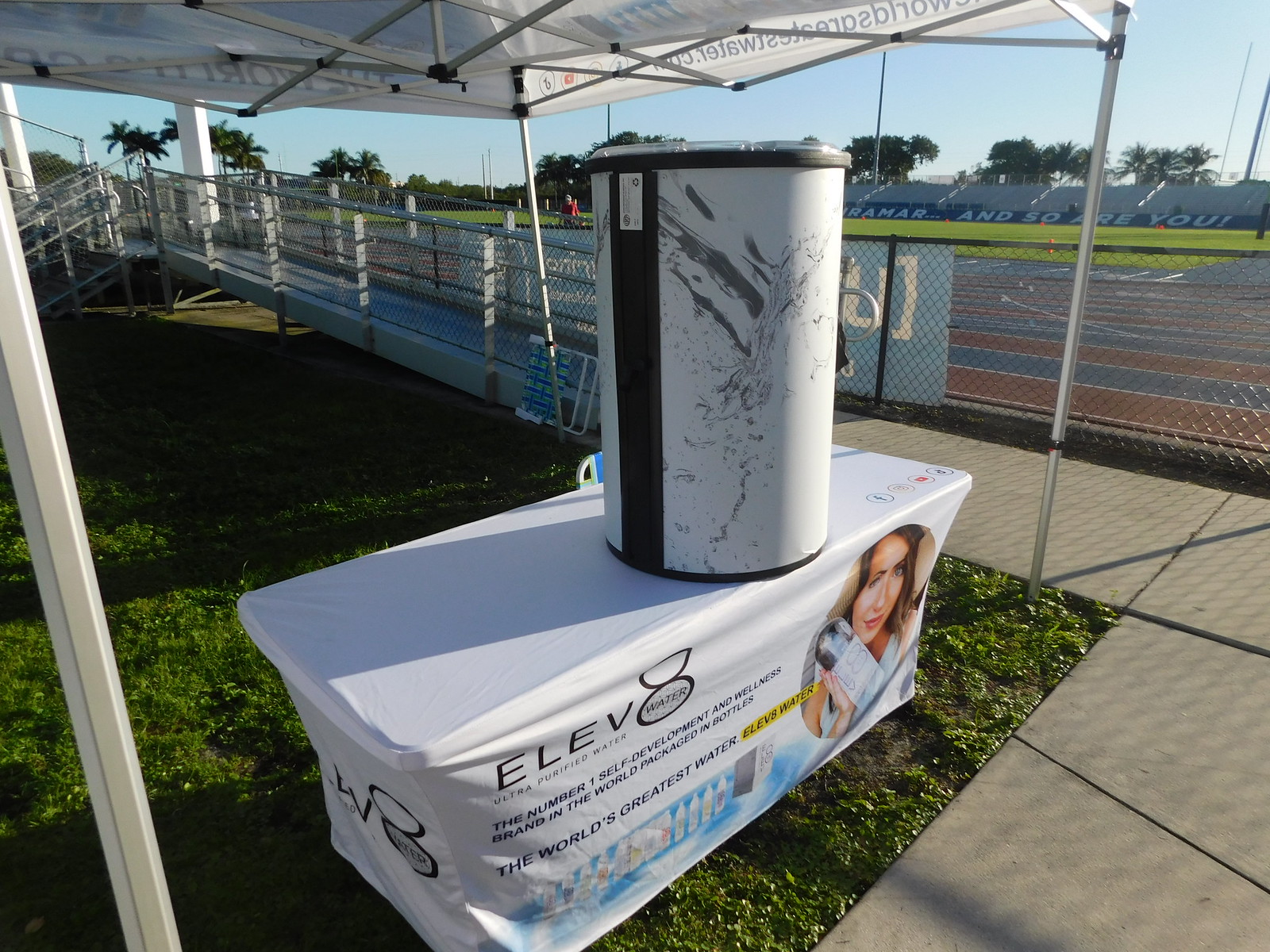The image depicts a promotional setup for Elevate Water, featuring a table adorned with a branded tablecloth showcasing an advertisement that includes a woman holding a bottled water, and bearing the slogans "Ultra Purified Water," "The World's Greatest Water," and "The Number One Self-Development and Wellness Brand in the World." On the table, positioned under a collapsible canopy with matching branding, rests a white and black barrel, likely used as a cooler. The backdrop reveals a large stadium, identifiable as an American football stadium by the visible goals and stands. The stands also display partial text that reads "RMR and so are you," although the entire phrase is cut off. The setting hints at both a sports and wellness theme, merging athletic elements with the brand's emphasis on purity and health.